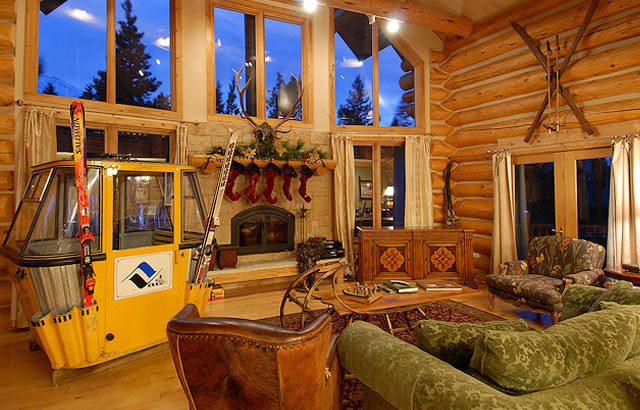This photorealistic image, possibly a real photo, captures an angled view of a cozy living room inside a rustic ski cabin made of light-colored wooden logs. Dominating the background is a tall wall of windows that bathe the room in natural light, revealing the tops of triangular pine trees and a blue, dusk sky. In the center of the room stands a fireplace adorned with stockings on a light wood mantle decorated for Christmas, complete with an antler head. To the left of the fireplace, there is a charming enclosed yellow ski gondola featuring a red and white ski on its exterior, adding a whimsical touch. The bottom right corner showcases a comfortable seating area with a green fabric couch, a coffee table, and a distinguished brown leather wingback chair with nailhead trim. Nearby, a floral chair adds a splash of color to the warm, inviting space.